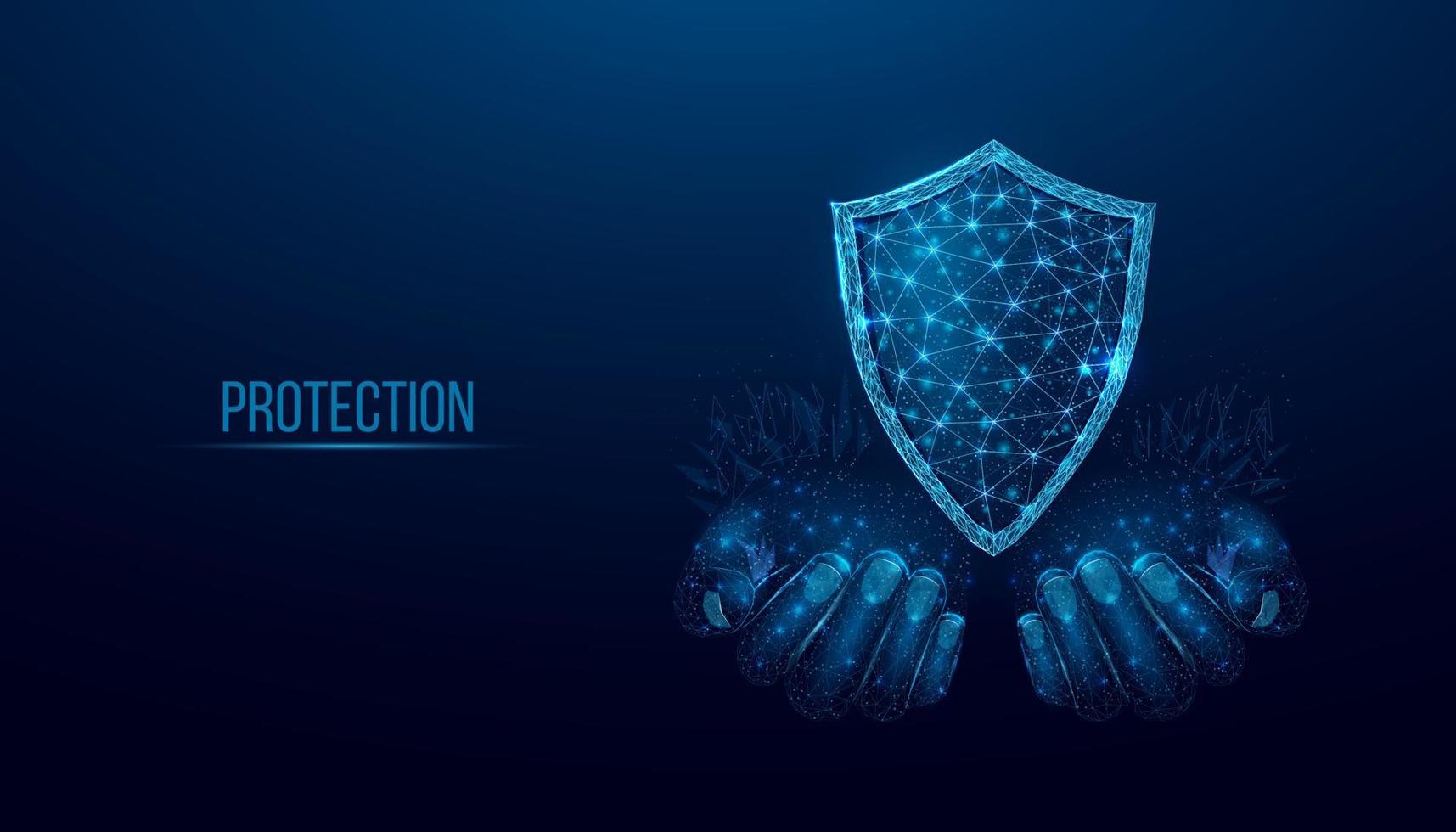This detailed illustration predominantly features a blue color palette, with a gradient background that transitions from dark blue at the bottom to lighter blue at the top. Central to the image are two slightly transparent hands, in shades of steel blue and light blue, positioned palms up as if to hold something. Hovering just above the hands is a light blue shield, which is outlined with a thick border and tapers into three points at the top and one at the bottom. The shield's internal surface is adorned with a glowing line grid of triangular patterns, created by interconnected light blue dots that evoke the appearance of a star constellation. To the left of the hands and shield, the word "Protection" is prominently displayed in blue text, with an underline for emphasis. The stylized design and the celestial elements of the shield suggest a theme of cybersecurity and protection, portraying an advanced and interconnected system designed to safeguard against digital threats.